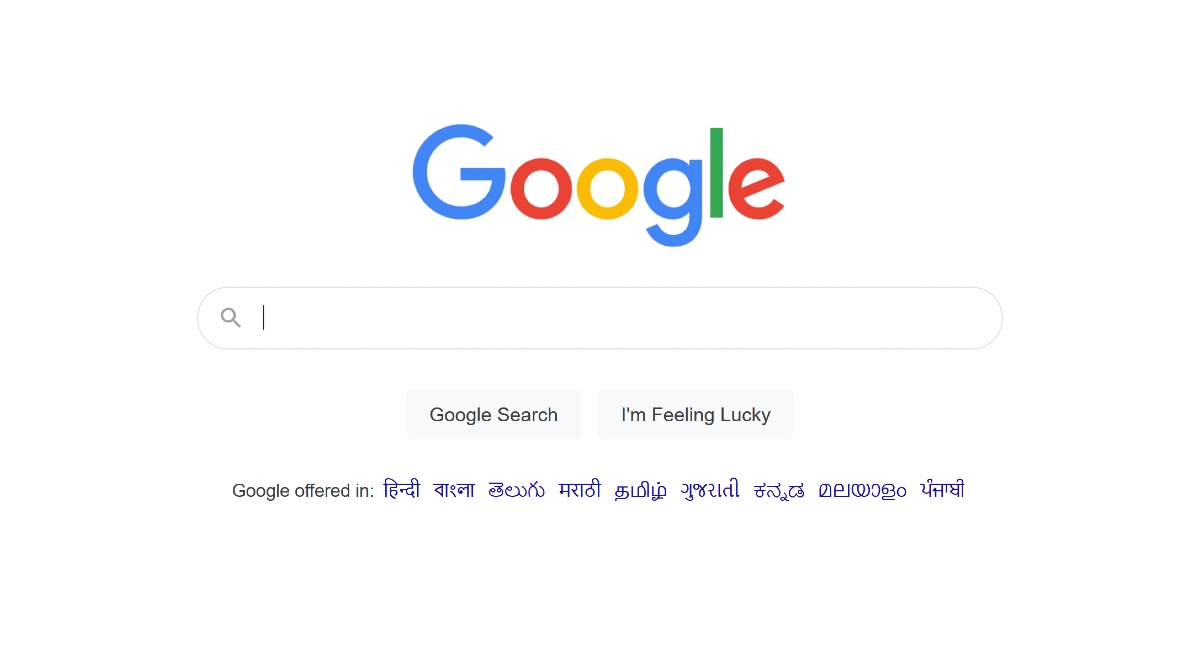This image is a screenshot of a Google search page, featuring a clean and minimalistic design on a crisp white background with no borders. At the top center of the image, the Google logo is prominently displayed, with each letter in its iconic colors: a blue 'G', a red 'o', a yellow 'o', another blue 'g', a green 'l', and a red 'e'. Below the logo sits the familiar search bar, outlined by a thin gray line, with a gray search icon positioned at the left end and a vertical blinking cursor line inside the bar.

Immediately beneath the search bar are two buttons: the "Google Search" button on the left, and the "I'm Feeling Lucky" button on the right. Both buttons feature black typeset against a gray background.

Toward the bottom of the image, the text "Google offered in" is displayed in very small black font, accompanied by a series of small purple characters that appear to be in Arabic or another language, indicating language options available for the user. The overall layout and color scheme reflect Google's characteristic simplicity and user-friendliness.